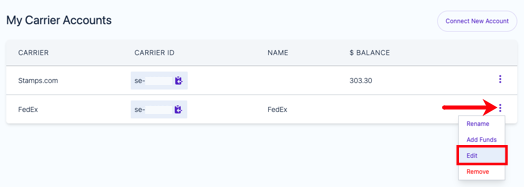This image is a screenshot of a user interface titled "Carrier Accounts". In the top left corner, the header "My Carrier Accounts" is displayed, while the top right corner features a "Connect New Account" button illuminated in purple, inviting users to add a new account.

Below the header, a table is organized with the following columns: "Carrier", "Carrier ID", "Name", "Balance", and "Actions". The first row in the table lists "stamps.com" under the "Carrier" column, displaying "SC-" as its Carrier ID and showing a balance of "$303.30".

Adjacent to this row, a battery icon with an arrow pointing left is possibly representing some status indicator. The next row lists "FedEx" as the Carrier, which has no balance under its "Balance" column. On the far right of the FedEx row, there are three vertical ellipses, indicating a menu that, when clicked, offers options such as "Rename", "Add Funds", "Edit", and "Remove".

Overall, the visual layout appears user-friendly and organized, intended to facilitate the management of various carrier accounts for the user.